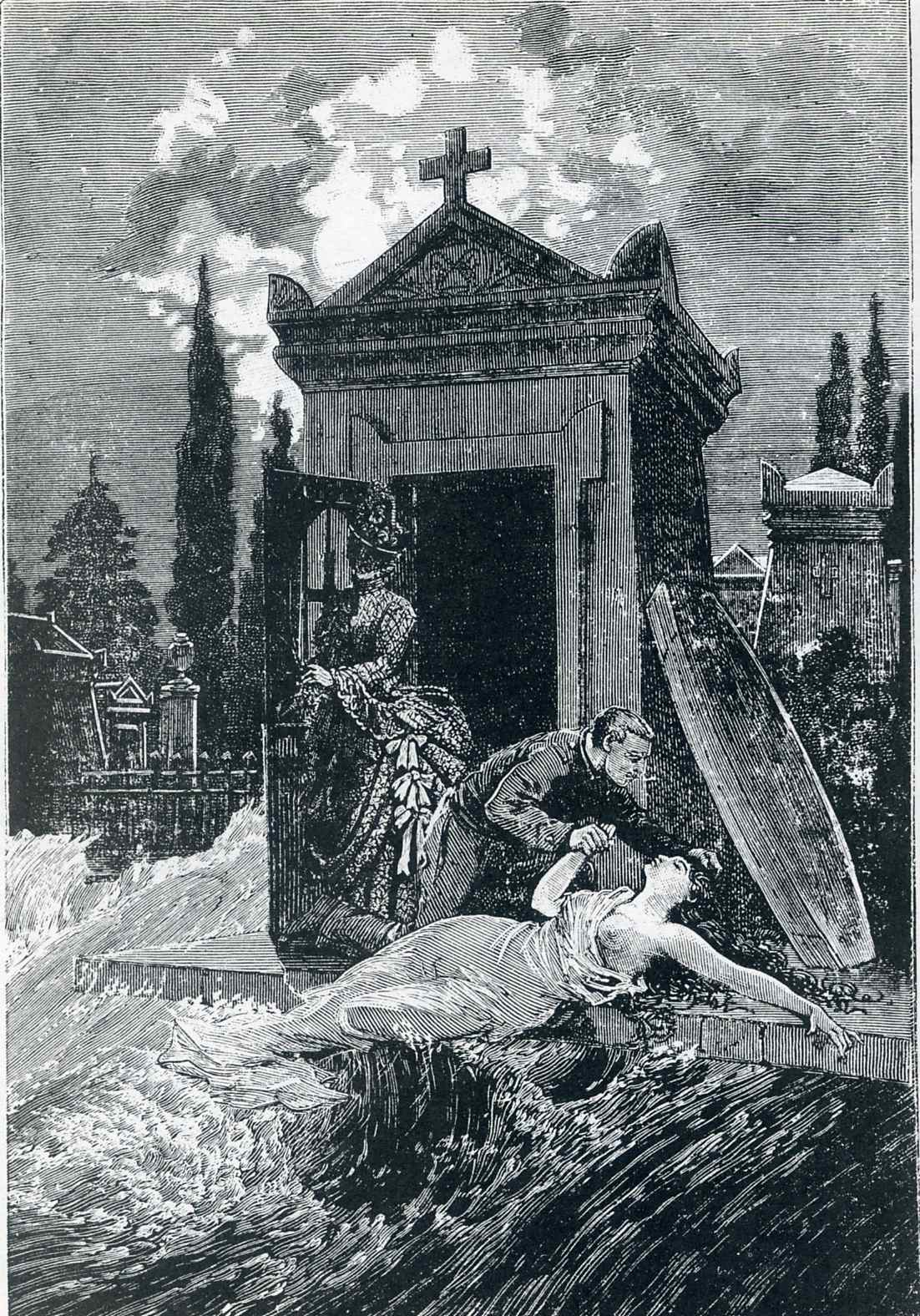The image depicts a detailed black-and-white drawing of a graveyard, centered around a small stone mausoleum with a triangular roof topped by a cross. Waves of water are crashing at the base of the scene. The mausoleum's door, which faces the front, is ajar and has four glass panels. Leaning against the mausoleum is a coffin lid.

Next to the door stands a woman in a Victorian dress and veil, her attire hinting at nobility. To the right, a man with short hair and dressed in a shirt is kneeling, grasping the hand of a woman lying on the ground. The woman, who appears to be faint or unconscious, has her left arm extended outward and her head raised slightly towards the man, who looks worried.

In the background, the graveyard extends with additional mausoleums, gravestones of various shapes, and scattered trees. A fence can be seen among the tombstones. The sky is filled with clouds, sketched in different shades, adding depth to the scene.